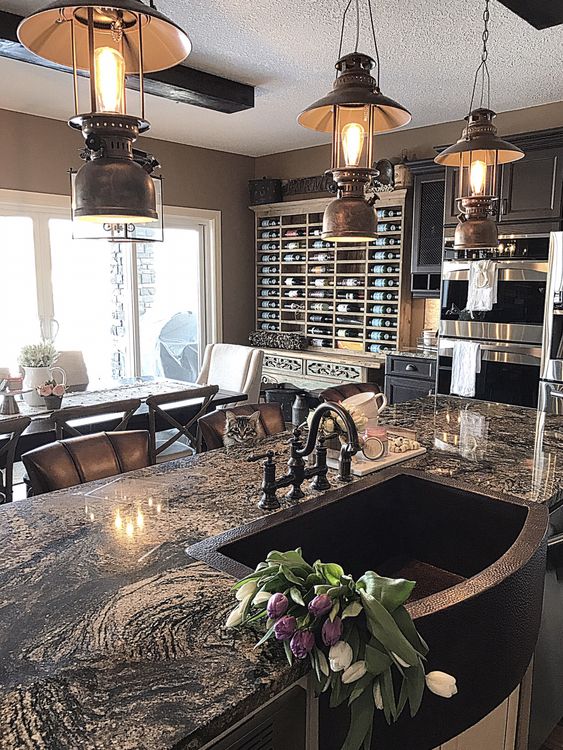This interior photograph showcases a spacious and well-appointed kitchen. At the center of the image, a large kitchen island with a sparkling gold and black granite countertop prominently stands out. The island features a deep, brown sink with a curving front that integrates seamlessly into the rectangular shape of the island. The sink contains a mix of white and purple tulips, their stems drooping and the petals showing signs of wilting.

Above the island, three elegant, vintage-style lanterns are suspended, providing warm illumination to the kitchen. To the right of the island, a trio of barstools awaits, with a curious little cat perched on the middle seat, gazing into the camera. 

The kitchen's color palette leans towards muted beige and brown tones, offering a cozy and inviting atmosphere. In the background, a window allows sunlight to flood the space, although the light outside is somewhat overexposed. Below the window, a generous wine rack lines the back wall, stocked with numerous bottles, hinting at a well-curated collection.

Further details include sleek stainless steel appliances, such as a partially visible refrigerator and a black stove with stainless accents. A dining table with chairs is positioned near the island, adorned with a small vase of flowers, enhancing the room's warm, homely ambiance. Various kitchen essentials, including teacups and trays, are neatly arranged on the counters, contributing to the overall functionality and charm of this beautiful room.